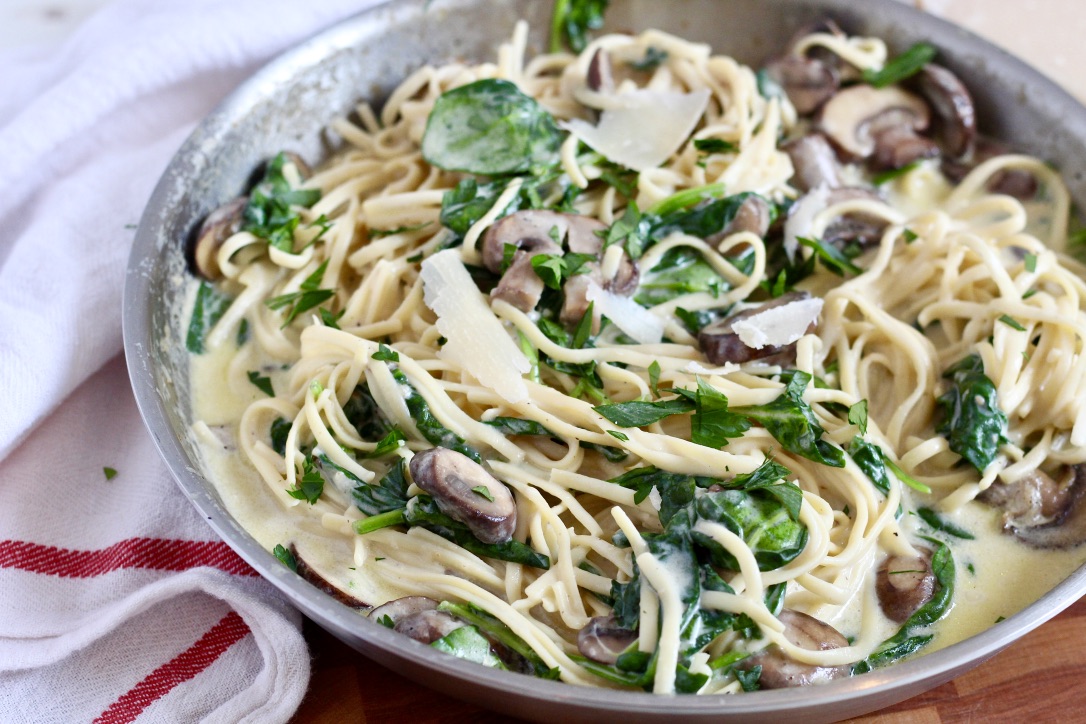A vibrant landscape-oriented color photograph showcases a culinary delight, centered on a silver metal dish that straddles the line between a shallow bowl and a plate. The dish rests elegantly atop a brown wooden surface, accompanied by a white napkin with a striking red stripe on the bottom left corner. The main highlight is a sumptuous serving of pasta, possibly spaghetti or linguine, immersed in a creamy white sauce, nearly soupy in its richness. This decadent pasta is generously topped with an array of green vegetables, likely spinach, and interspersed with cooked greens, enhancing the visual and textural appeal. Adding to the feast are perfectly cooked mussels, scallops, shrimp, and possibly other seafood elements, creating a harmony of flavors reminiscent of a bouillabaisse. Grated Parmesan cheese and chopped mushrooms are sprinkled liberally over the dish, adding an earthy richness that complements the creamy sauce. This meticulous presentation exemplifies photographic realism, capturing the essence of gourmet food photography.